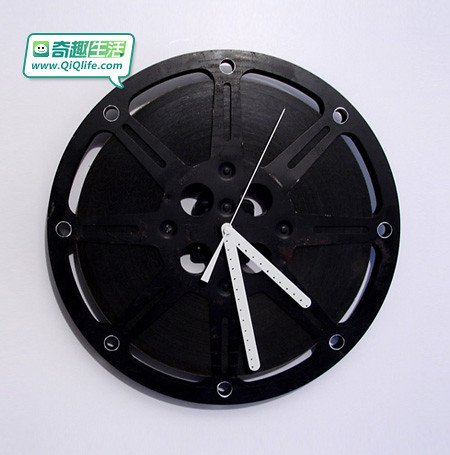Displayed against a pristine white wall, this unique clock features a design reminiscent of intricate gearwork. The clock's structure brings to mind a car's rim, with matte black, flat-painted elements similar to brake rotors visible behind the primary frame. The exterior frame, resembling wheel spokes, has evenly drilled holes that serve as markers for the clock's hours. The clock hands, striking in bright white, indicate the time for minutes, hours, and seconds with clear precision. Adding a touch of whimsy, a small text bubble with a smiley face is positioned in the upper left corner, bearing the website "www.QIQLife.com". This combination of industrial design elements with playful details creates a captivating and functional piece of decor.